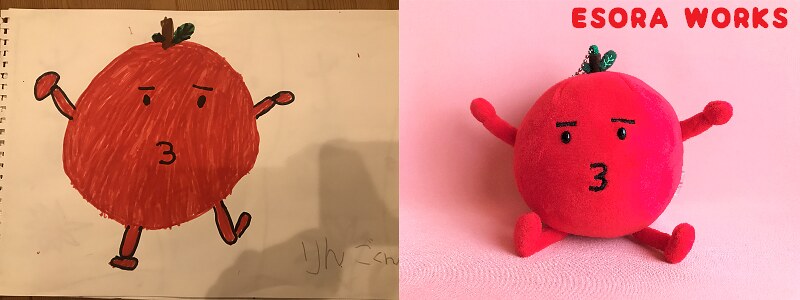This image consists of two distinct parts placed side by side. On the left, there is a hand-drawn sketch, while on the right, there is what appears to be a photograph or a digitally created version of the same subject. Both images depict a charming, anthropomorphic tomato-like creature characterized by a round red body, two arms, and two legs. The character's face features two small dot eyes, with straight lines above them, and a mouth shaped like the number three. Atop its head are small leaves, suggesting it is indeed a tomato.

The right-hand side image, which resembles a photograph, has a label at the top reading "E-S-O-R-A, Works." The left-hand sketch appears to be a recreation of this photograph. Despite a few lumps and uneven strokes, the hand-drawn rendition captures the essence of the photographed character quite well, including the distinctive three-shaped mouth, leaf-topped head, and overall form. The drawing, seemingly done by a novice or a child, is signed in the corner and made on unlined white notebook paper. The resemblance between the two images highlights the effort and attention put into replicating the original work.